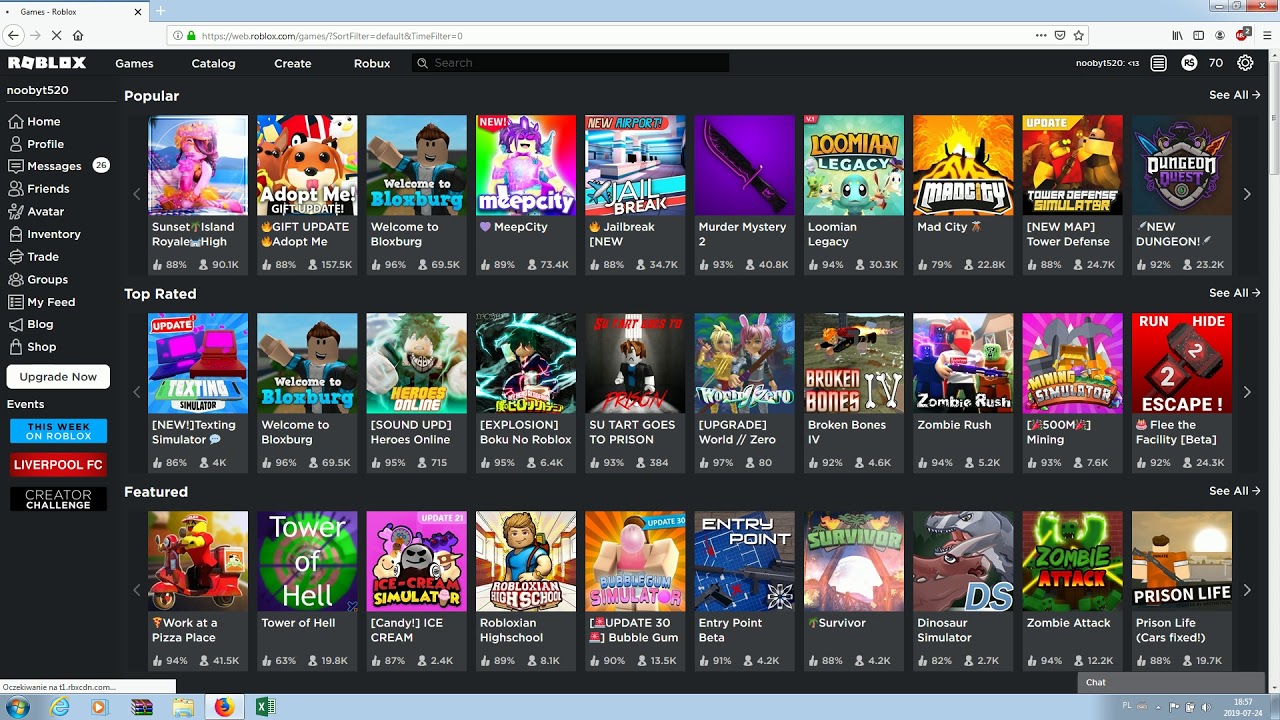This image is a detailed screenshot of the Roblox website's "Games" tab, captured on a device running Windows 7. The familiar Roblox name and logo can be seen prominently in the top left corner, confirming the website. The central portion of the image showcases a selection of popular games available on Roblox, including titles such as Summer Island, Sunset Island, Royal High, Adopt Me, Welcome to Bloxburg, Meep City, and Jailbreak. On the left side of the screen, various navigation tabs are visible, such as Home, Profile, Messages, Friends, Avatar, among others. Additionally, the screenshot includes the Windows taskbar at the bottom, with the classic Windows 7 logo in the bottom left corner, indicating the operating system. The browser in use appears to be Mozilla Firefox, adding a layer of context to the browsing experience.